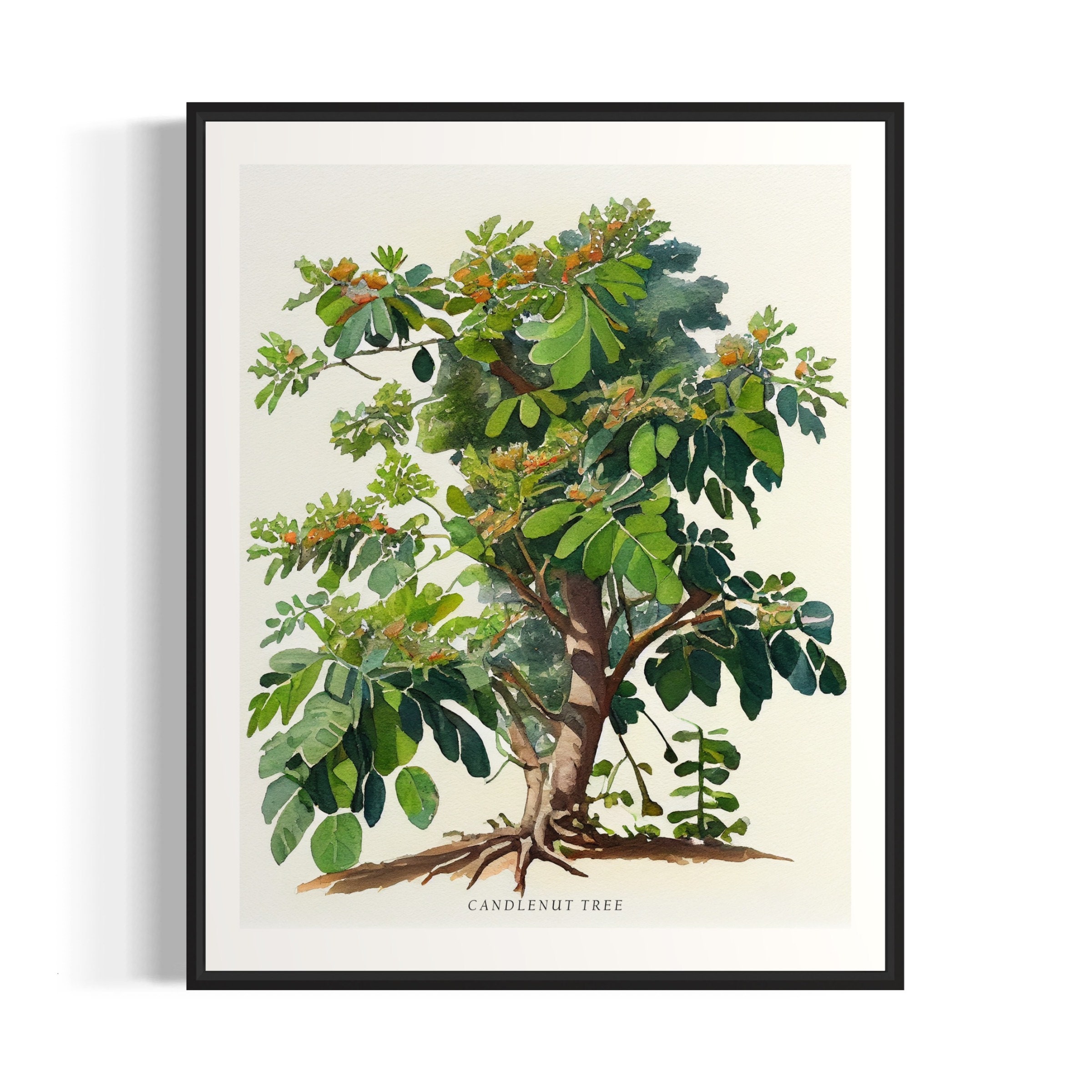This is a detailed and professionally framed photograph of a painting depicting a Candle Nut Tree. The artwork, appearing to be done in a pencil or watercolor style, is set against a cream-colored background with a thick white matting and a thin black frame, casting a slight shadow on the left side. The tree, prominently displayed, features a thick brown trunk with sprawling green leaves and clusters of small orange flowers. Below the tree, the brown ground is visible, depicting roots and a small sapling growing at the base. The name "Candle Nut Tree" is inscribed at the bottom of the painting in small black letters. The photograph emphasizes the intricate details, including the texture of the leaves and flowers, giving a realistic and slightly cartoonish appearance to the tree. The shadows and framing suggest a professional setup, highlighting the natural beauty and structure of the Candle Nut Tree.